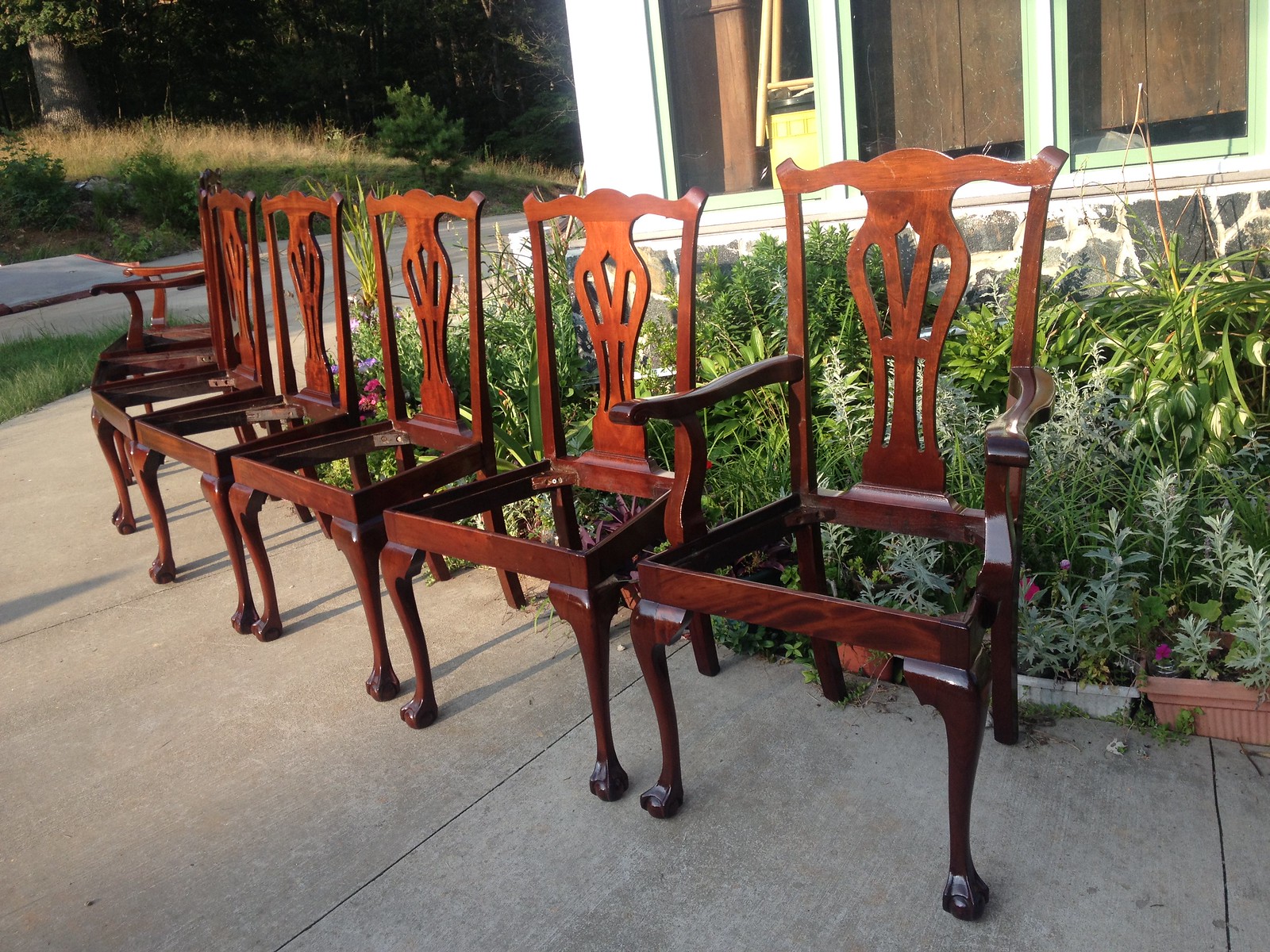This photograph, taken outside either a home or business at sunrise or sunset, features a striking arrangement of seven ornate, antique wooden chair frames lined up along a cement walkway. The walkway, which curves aesthetically around the building, is flanked by a small planted garden with lush green plants both in the ground and in planters. Each chair, crafted from dark wood, boasts an elegant and decorative wooden back, though they lack seats and upholstery. The two chairs anchoring the row have arms, while the four in the middle do not. The background reveals a building with a stone foundation and white walls, punctuated by three large picture windows that appear partially obstructed by cupboards, adding a quaint, rustic charm to the scene.